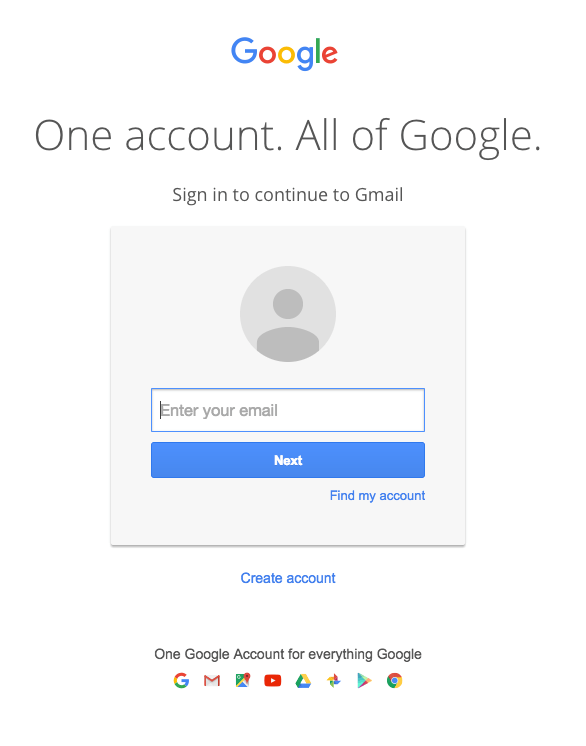This image is a screenshot of a Google account sign-in page. At the top center, the iconic Google logo is prominently displayed in red, yellow, green, and blue lettering. Directly beneath the logo, bold black text reads "One account. All of Google." In smaller black text below this, it states "Sign in to continue to Gmail."

Central to the image is a large light gray square containing a gray circle filled with a silhouette of a person, representing the user profile picture. Below this avatar, there is a white text bar labeled "Enter your email," intended for user input. Situated beneath this text bar is a blue "Next" button. Towards the lower right of the "Next" button, the link "Find my account" is visible.

At the bottom edge of the light gray square, light blue text prompts "Create account." In smaller black text below this, it reassures users with the statement "One Google account for everything, Google." Surrounding this statement are various logos representing different Google services and products, such as Gmail, Search, Maps, YouTube, Google Drive, and Google Chrome.

The background of the screenshot is a plain white, providing a clean and uncluttered look. The image itself has a vertical rectangular orientation, emphasizing the tall layout of the sign-in page elements.